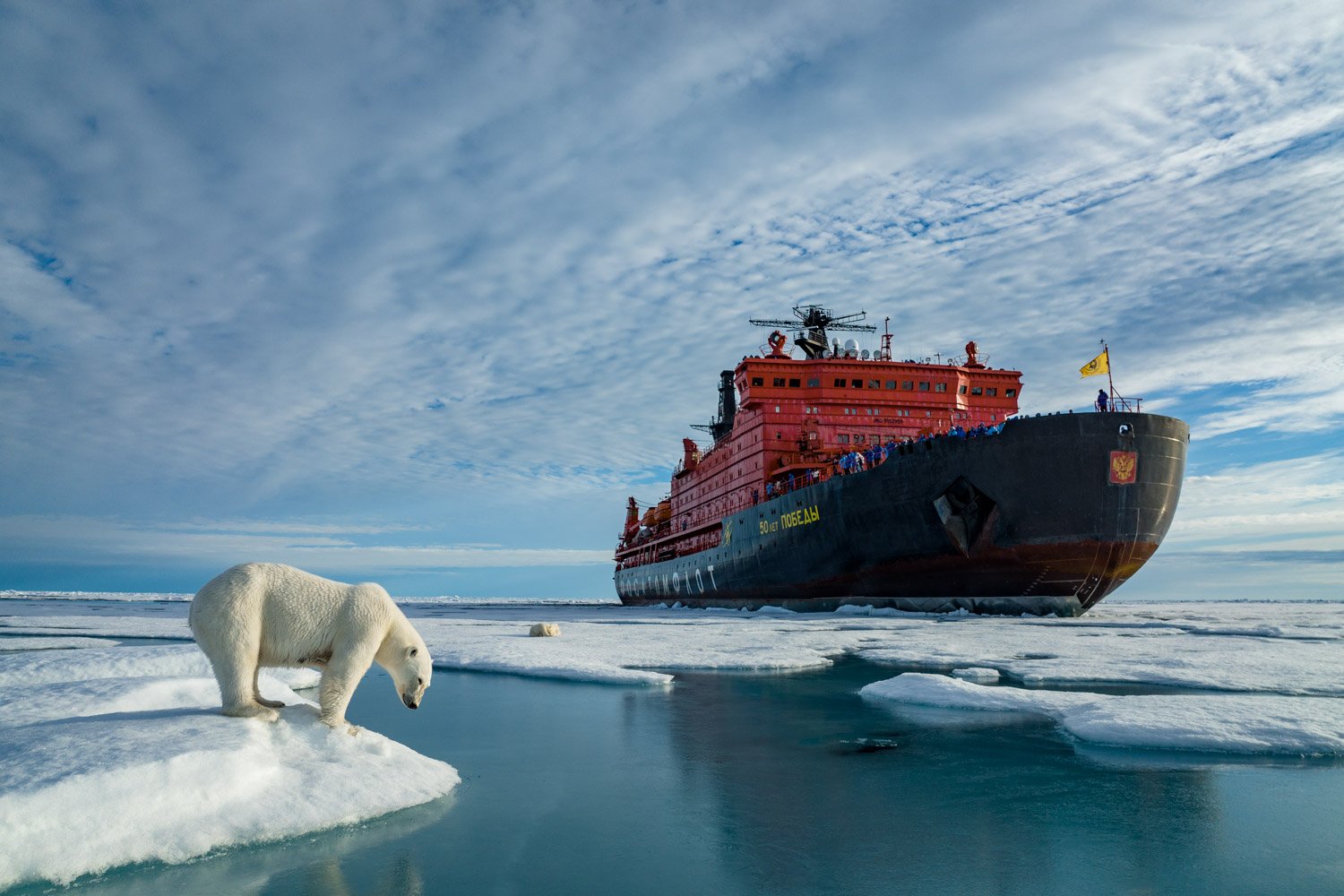This color photograph captures a poignant Arctic scene where a massive ship, primarily black with a red top, named Togose (partially obscured), dominates the right side of the frame. The ship is navigating through a patchy ice field, breaking up the ice, and creating a stretch of calm, open water. At the forefront, on a piece of ice to the left, stands a lone polar bear, appearing thin and forlorn, gazing down into the water. The bear is in profile, allowing a clear view of its body and a wistful expression on its face. Closer inspection of the ship reveals a yellow flag at the bow and various power antennas atop the structure. The sky above is predominantly blue, dotted with comprehensive white clouds. In the distance, amidst the fragmented ice, a faint shape suggests the possibility of another polar bear, curled up and possibly asleep, adding to the remote and desolate atmosphere of the scene.